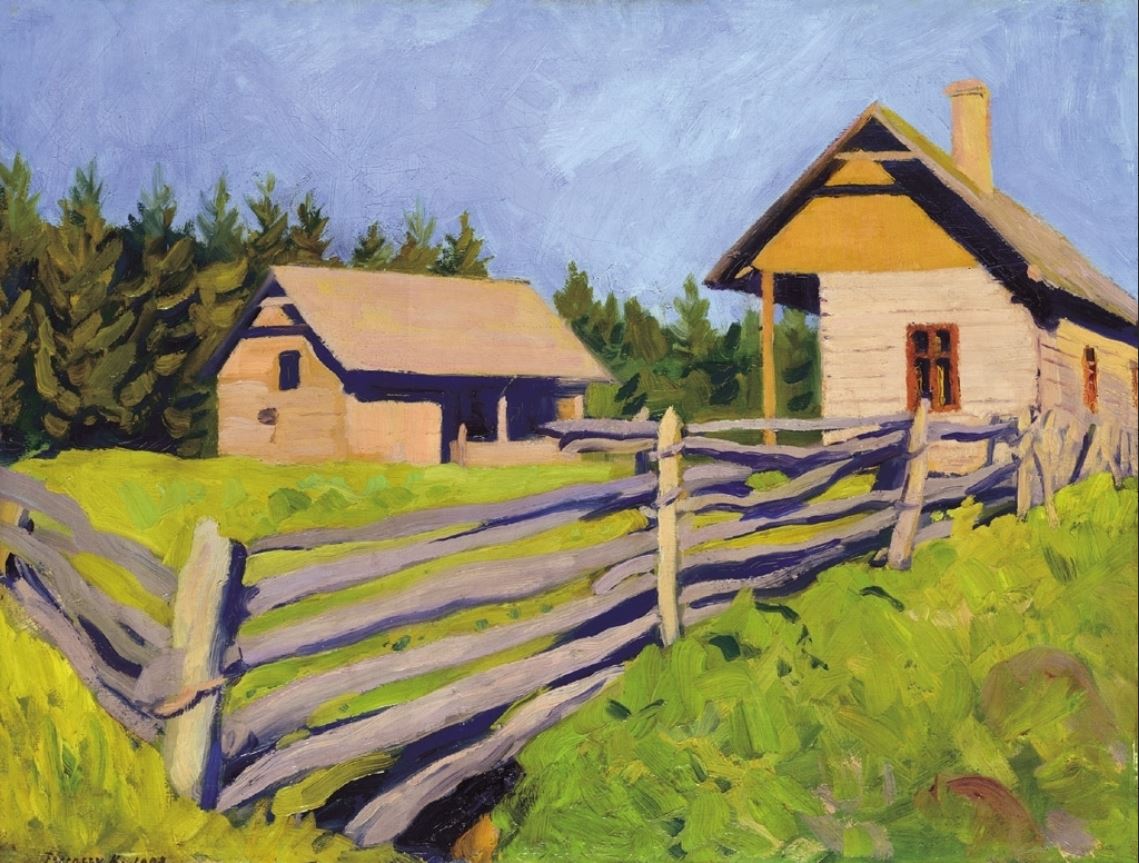This detailed oil painting, titled "Bowery N. Guttini" by artist Ferenczy Karoly, created in 1908, depicts a charming rural scene with two distinct buildings set in a lush, green field surrounded by a weathered, wooden split rail fence. The property features a fenced area with five horizontal wood posts paralleling the image, some parts appearing to fall apart. The house on the right is a log cabin with an A-frame roof, adorned with mustard-colored gables, red window trim, and a chimney of light brown. It includes support braces at the peak and has a quaint porch supported by two sturdy 4x4 posts. Across the field stands a shed with a simple beige facade and an A-frame roof, also featuring a support brace and a single cutout window. This structure lacks a chimney and is more simplistic in design compared to the house. The landscape is adorned with high greenery, suggesting overgrown grasses or shrubs, and is framed by a thick stand of pine trees that encircle the scene. Above, the sky is a serene light blue, adding to the tranquil, pastoral setting captured in the modern Impressionist style of the painting.